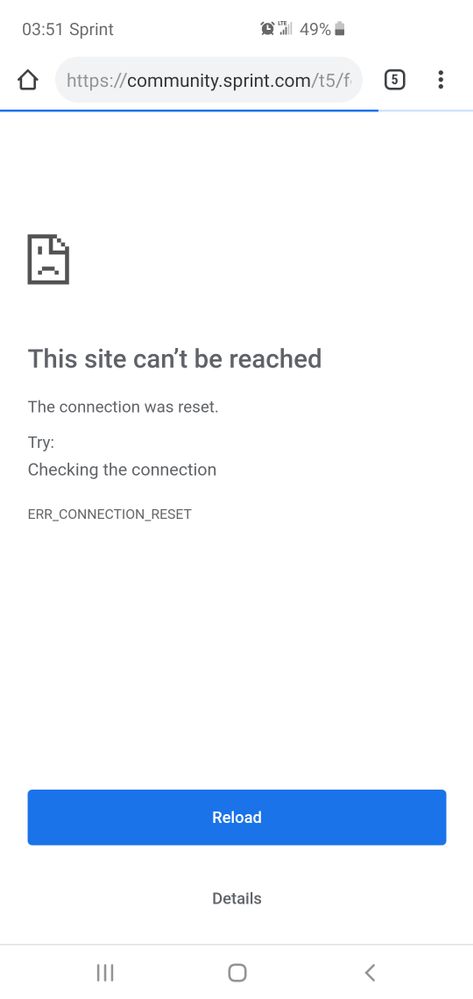A screenshot of a smartphone displaying a "Site can't be reached" error on a web page. At the top left corner, the time reads 3:51, with the word 'Sprint' next to it. In the upper right corner, icons for an alarm, cell phone reception, and a battery at 49% are visible. Below that, the web address in the browser's address bar reads "https://community.sprint.com/T5/F." To the left of the address bar is a home button, while to the right is a symbol indicating multiple tabs open (five tabs). The main content area of the screenshot shows a message that reads "This site can't be reached. The connection was reset. Try checking the connection." At the bottom center, there are two buttons: one for reloading the page and another labeled "Details."